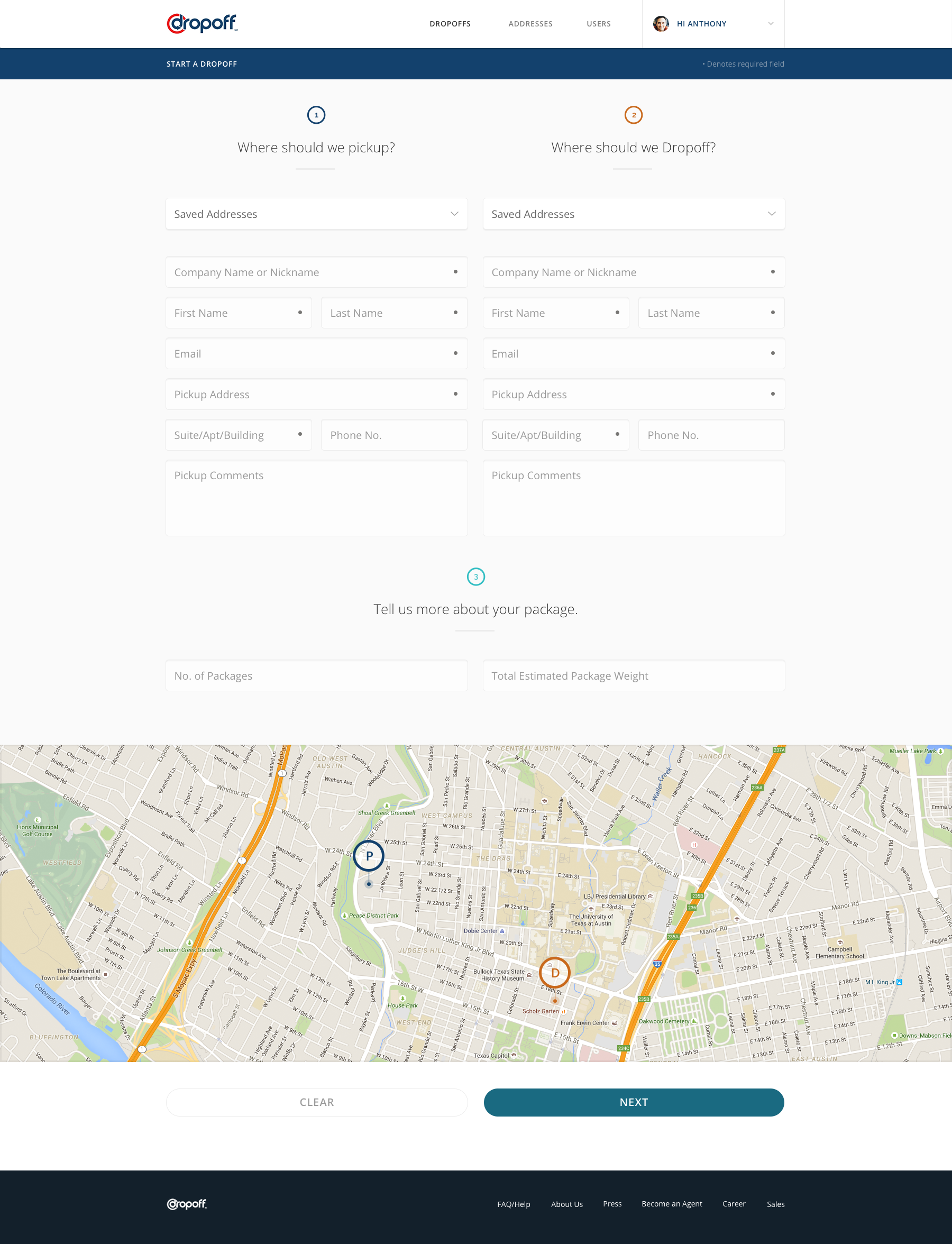The image features a white background with a "Drop Off" label in the upper-left corner. Towards the top-right, there is a cluster of blurred text and three clickable areas of unknown labels. Adjacent to these clickable areas is a profile picture. Beneath the top section is a dark blue horizontal line containing some illegible text. 

Just below this line, there are two notable circles: a blue circle with text under it and a red circle with text under it. Associated with these circles are several dropdown menus, though their options are unclear. Further down, there are multiple text boxes intended for user input.

Centrally placed on the image is a light blue circle, again with text underneath it. Directly below the central blue circle, a map is displayed, featuring a couple of pinpoint location markers. At the bottom of the image, there is a "Clear" button positioned to the left, with a blue button adjacent to the right.